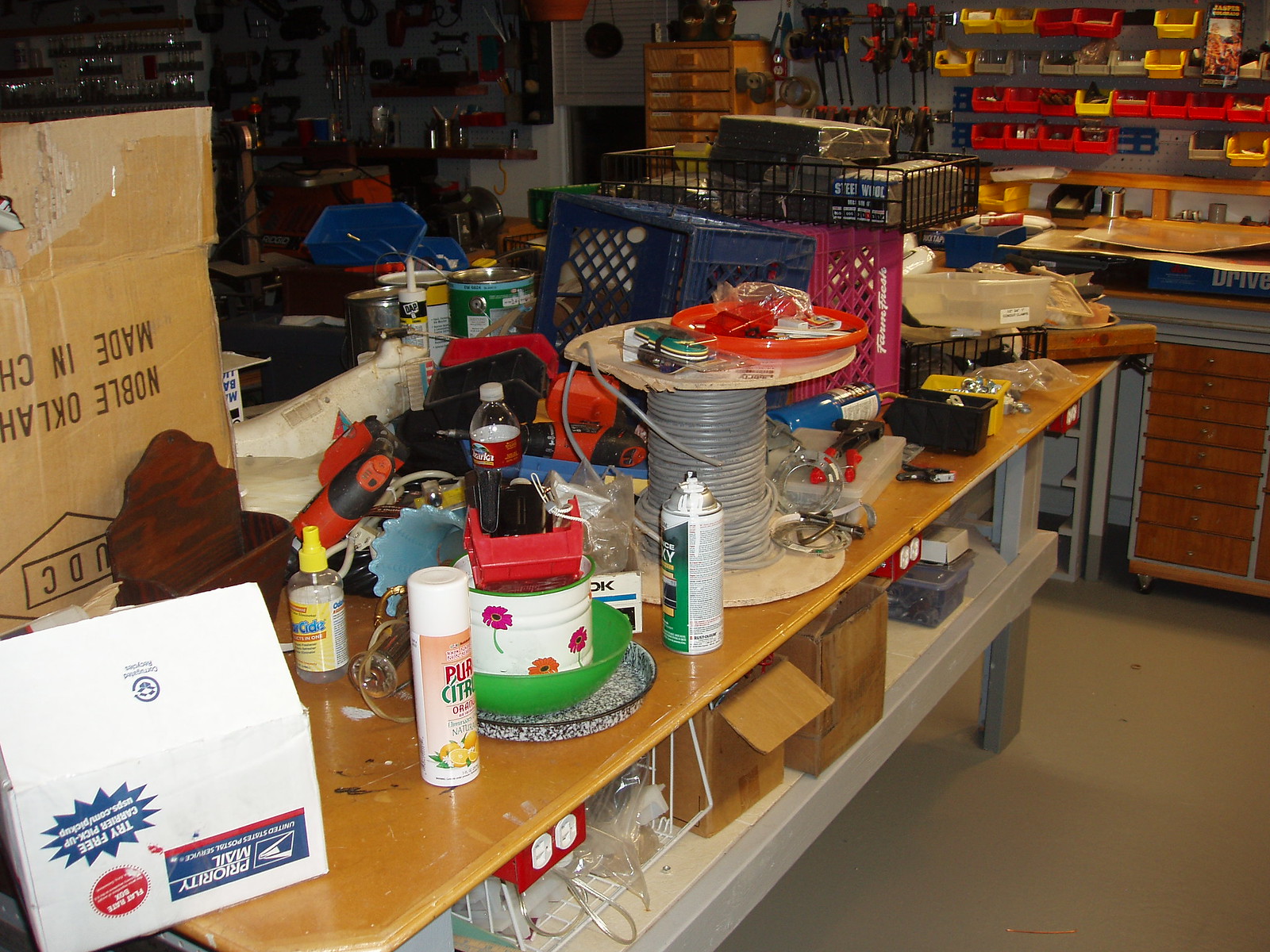The image depicts a cluttered interior, possibly a hardware store or a public garage. Dominating the scene is a brown wooden countertop, heavily laden with various items. At the far left sits a white Priority Mail box adorned with red, white, and blue lettering. In front of that, there is a large brown box.

A dark brown wooden shelf is also visible, holding an assortment of objects including a red drill, a clear bottle with a yellow top, and a white aerosol can with a cap. Nearby, a green bowl nests within a white tin bowl decorated with flowers, and an uncapped aerosol can stands next to a half-empty clear bottle of brown liquid, perhaps soda.

A large wooden spool wrapped with gray wire lies in the vicinity, accompanied by a blue and red plastic crate. Additionally, a small black wire shelf is filled with various boxes.

The back wall, painted gray, is lined with shelves, their contents indeterminate from the image. Towards the front, a wooden counter is piled high with cardboard materials. This area features small red and yellow plastic inserts designed for tool storage.

Below the counter, multi-drawer cabinets rest on a beige floor. Further below the cluttered shelf area, there are more boxes and a beige wire shelf. The setting includes multiple red outlets with two white plug areas each, and near one outlet, there is a clear box containing silver items, likely nails or small tools. Overall, three red outlets can be seen within the image.